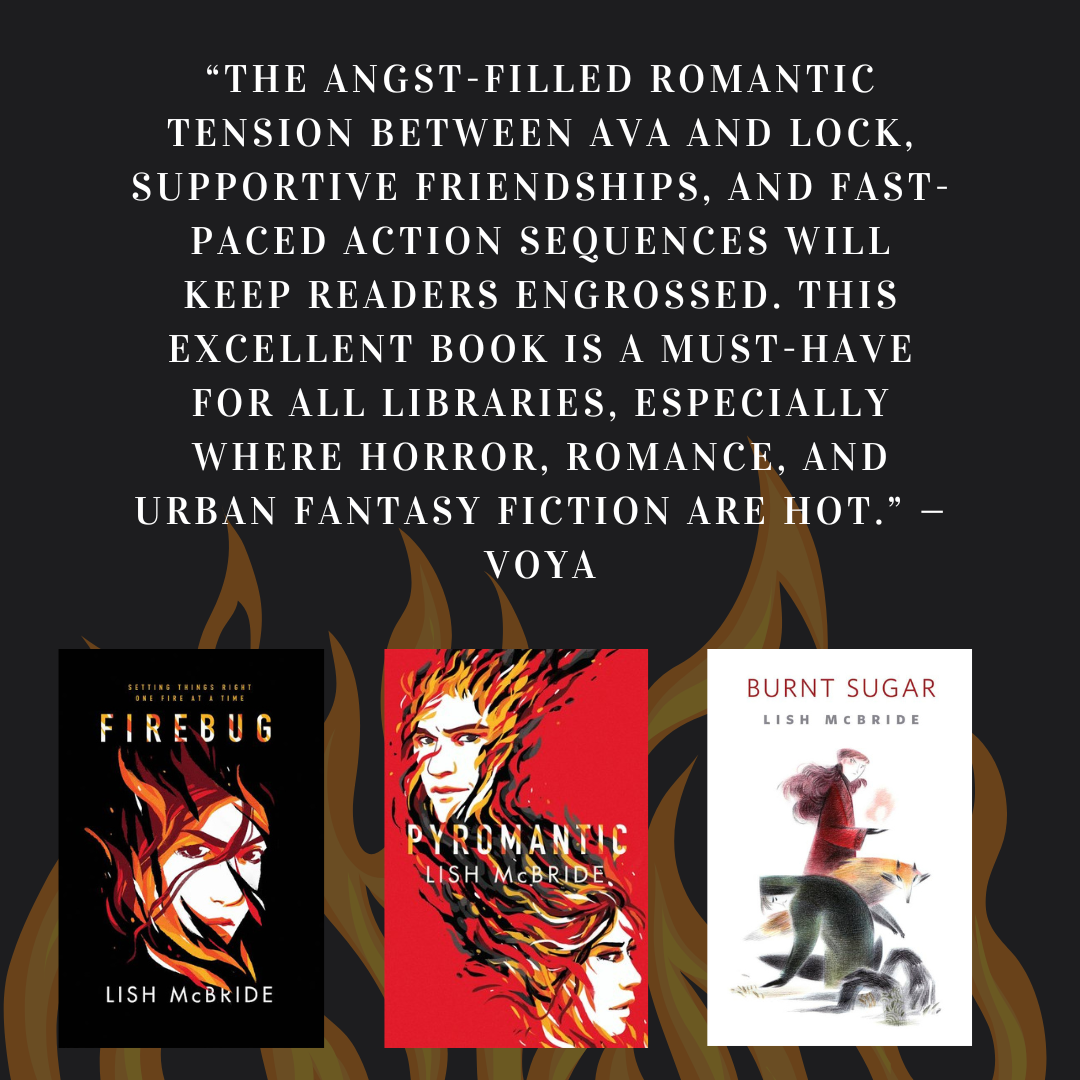Against a black background with rising orange flames at the bottom, the image prominently features the covers of three books by Lish McBride. At the top, a white-text quote reads, "The angst-filled romantic tension between Ava and Locke, supportive friendships, and fast-paced action sequences will keep readers engrossed. This excellent book is a must-have for all libraries, especially where horror, romance, and urban fantasy fiction are hot." — VOYA. 

On the left, the book titled "Firebug" shows a woman's face surrounded by flames, with the tagline "Setting things right, one fire at a time." The middle book, "Pyromantic," has a red background with a burning face of a man at the top left and a woman's face at the bottom right. Finally, the book on the right, "Burnt Sugar," depicts a human figure with a flame over his hand, alongside a fox and another human figure kneeling down.